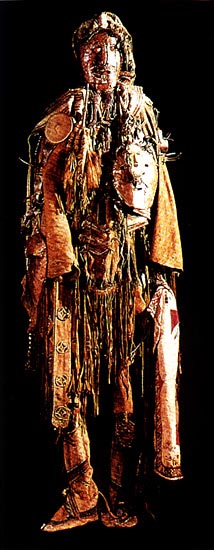This color photograph features a mannequin or model dressed in an elaborate ceremonial costume, set against a stark black background, likely showcased in a museum. The outfit, which predominates in shades of brown and gold, includes a goldish cap with a flap that drapes down the right side of the head. The face is obscured by a gold-colored mask, adding a macabre element to the attire. Around the neck, there is an ornate piece adorned with various hanging objects, some resembling giant coins or masks. A rounded shield or pad extends over the left chest, complementing a smaller round object on the upper right shoulder.

The ensemble behaves like an amalgamation of cloth and straw materials, with braided elements cascading down from the neck to the knee area. A brown leather belt cinches the waist, from which several stringy cloth pieces descend. Brown leather flaps hang from behind the shoulders to around the waist level, contributing to the outfit's extensive detailing. Additional components include a piece of white fabric on the left side, reaching nearly to the ankles, and a golden fabric with circular designs on the right, falling just below the knees. The mannequin's feet are fitted with brownish leather boots, completing the striking and intricate ensemble.